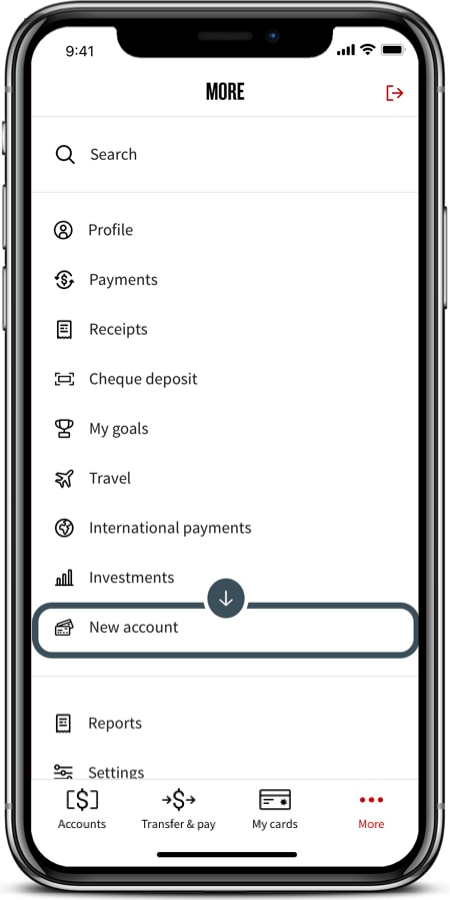The image features an iPhone displaying a banking or payment application on its screen. The timestamp in the top-left corner reads 9:41, and the device's status icons, including cellular signal, Wi-Fi connectivity, and a nearly full battery, are visible in the top-right corner. The app's interface has a clean, white background with the title "More" centered at the top, adjacent to a red box with a right-pointing red arrow, suggesting a navigational option to return to the previous screen.

Centrally displayed are multiple vertically aligned options related to banking and financial management, such as "Profile," "Payments," "Check Deposit," "Travel," "International Payments," "Investments," and "New Account." Notably, the "New Account" option is emphasized with a dark blue circle outline and an accompanying white arrow within a dark blue circle, indicating it is currently selected or highlighted. This suggests the image might be part of a tutorial or guide for creating a new account.

At the very bottom, the app offers a horizontal navigation bar with several clickable buttons labeled "Accounts," "Transfer and Pay," "My Cards," and "More," allowing users to easily navigate to different sections within the app. The overall presentation is clear, user-friendly, and purposefully guides the user through the account creation process.